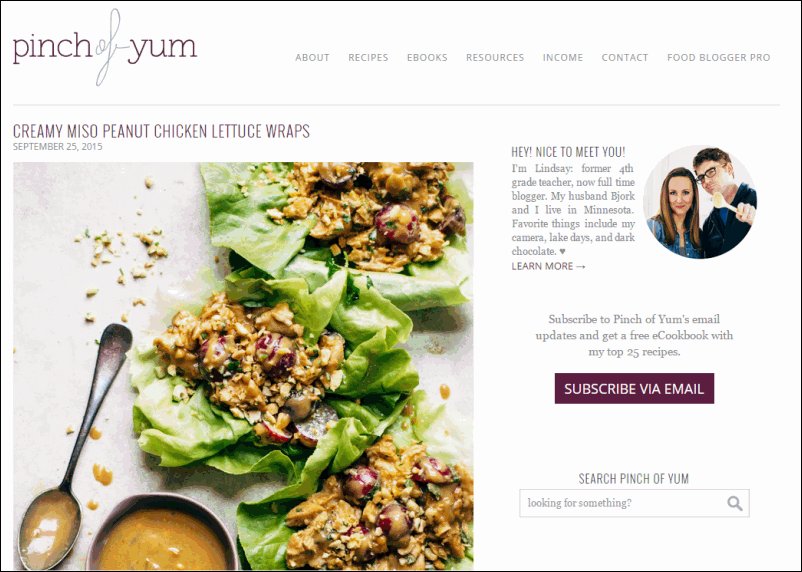On the "Pinch of Yum" website, which features a clean white background, the logo is prominently displayed in the upper left-hand corner. The word 'pinch' is written in lowercase plum-colored letters, 'of' is styled in a gray cursive font, and 'yum' is also in lowercase plum-colored letters. To the right of the logo, you'll find a navigation menu in uppercase gray text offering links to "Recipes," "Ebooks," "Resources," "Income," "Contact," and "Food Blogger Pro."

Displayed prominently on the page is a recipe titled "Creamy Miso Peanut Chicken Lettuce Wraps," written in uppercase plum-colored letters. This is followed by the publication date, "September 25th, 2015," in uppercase gray font. The majority of the page, approximately 60-75%, features a large, appetizing image of the lettuce wraps in the lower left-hand corner.

On the right side of the page, occupying around 30%, is a section with a circular thumbnail photo of Lindsay and her husband, Bjork, who run the website. This section greets visitors with the phrase, "Hey, nice to meet you!" in uppercase gray lettering, followed by a friendly introduction in regular sentence case: "I'm Lindsay, former fourth-grade teacher, now full-time blogger. My husband, Bjork, and I live in Minnesota. Favorite things include my camera, lake days, and dark chocolate ♥️." There is also a "Learn more" link with an arrow.

Below this introduction, visitors are invited to subscribe to Pinch of Yum's email updates and receive a free e-cookbook featuring the top 25 recipes. The subscription prompt is highlighted by a plum-colored block with the text "SUBSCRIBE VIA EMAIL" in uppercase white font. Following this, there's a search bar labeled "SEARCH PINCH OF YUM" in uppercase plum-colored letters, complemented by a magnifying glass icon to indicate search functionality.